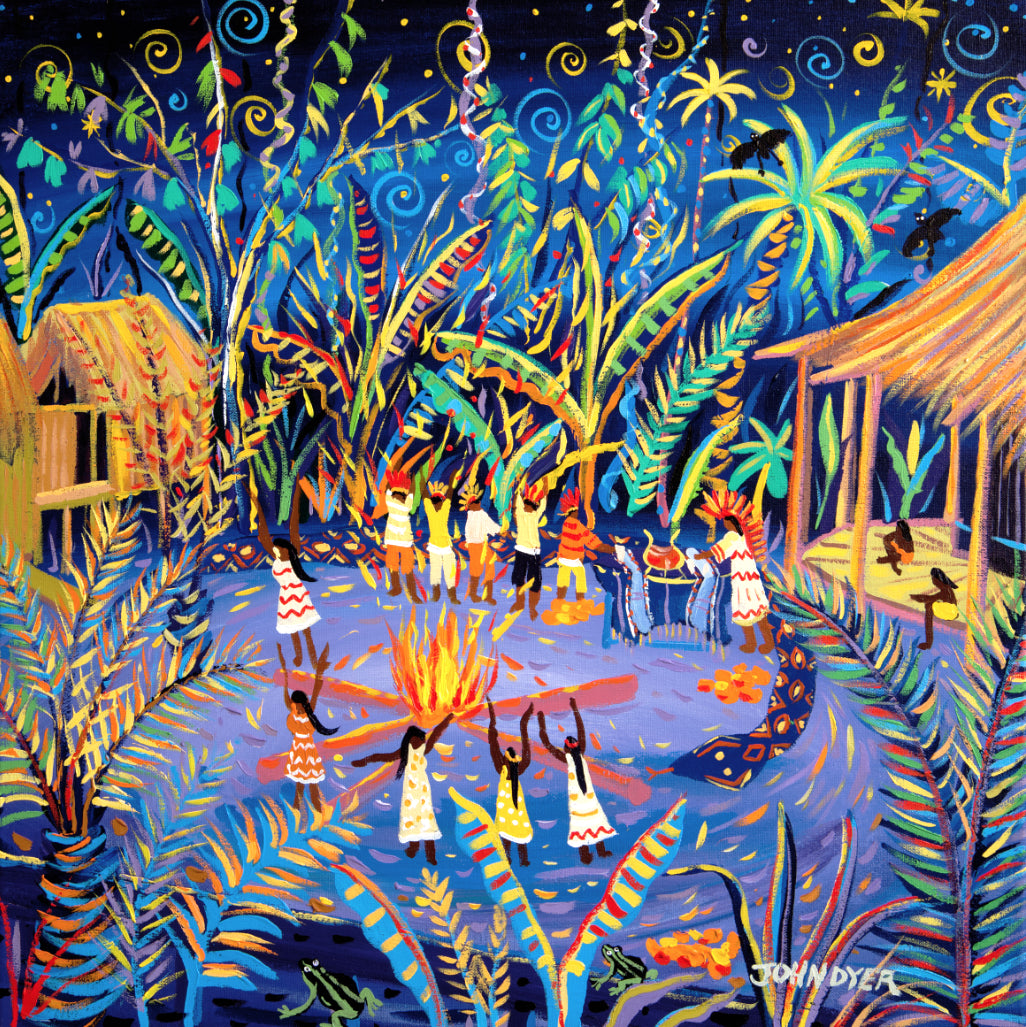This vibrant piece of artwork, signed by John Dyer in bold white letters in the bottom right corner, depicts a lively tropical celebration. At the center, a bonfire illuminates a colorful gathering of figures dressed in a variety of clothes and headwear, featuring hues like yellow, blue, red, and orange. Surrounding the bonfire are approximately ten individuals, some dancing and others in celebratory poses, with their hands up in the air. The scene is set against a lush, tropical backdrop with abundant greenery, including palm trees in striking colors of red, blue, and yellow. The sky is filled with dynamic swirls and curlicues, adding to the festive atmosphere. The setting includes two hatched-roof buildings—one on each side of the image—with a yellow and orange roof on the right. Frogs, dark silhouetted figures, and black birds enhance the whimsical nature of the scene. The background is enriched with shades of purple, further amplifying the artwork's vivid and spirited ambiance.